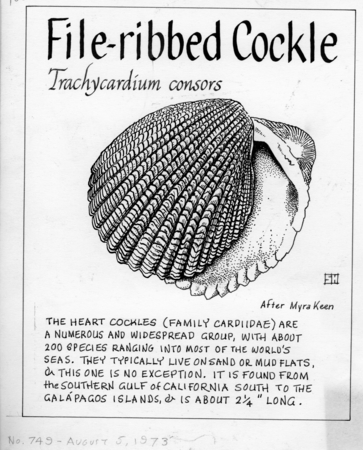This detailed caption describes an illustration of a file-ribbed cockle, scientifically known as *Trachycardium consors*. The illustration, reminiscent of old textbook illustrations, features a black and white image of the shell, showcasing both the top and bottom views. The shell resembles a clamshell with bumpy ridges covering its exterior and measures approximately 2 1/4 inches in length. Above the illustration, there is text identifying the shell's common and Latin names. The heart cockles, belonging to the family Cardiidae, comprise a numerous and widespread group with about 200 species found in most of the world's seas, typically residing on sand or mud flats. This particular species is found from the southern Gulf of California down to the Galapagos Islands. The text also includes a reference to the Marrakeen style and mentions an illustrator's signature on the right side, marking it as number 45, dated circa 1973.